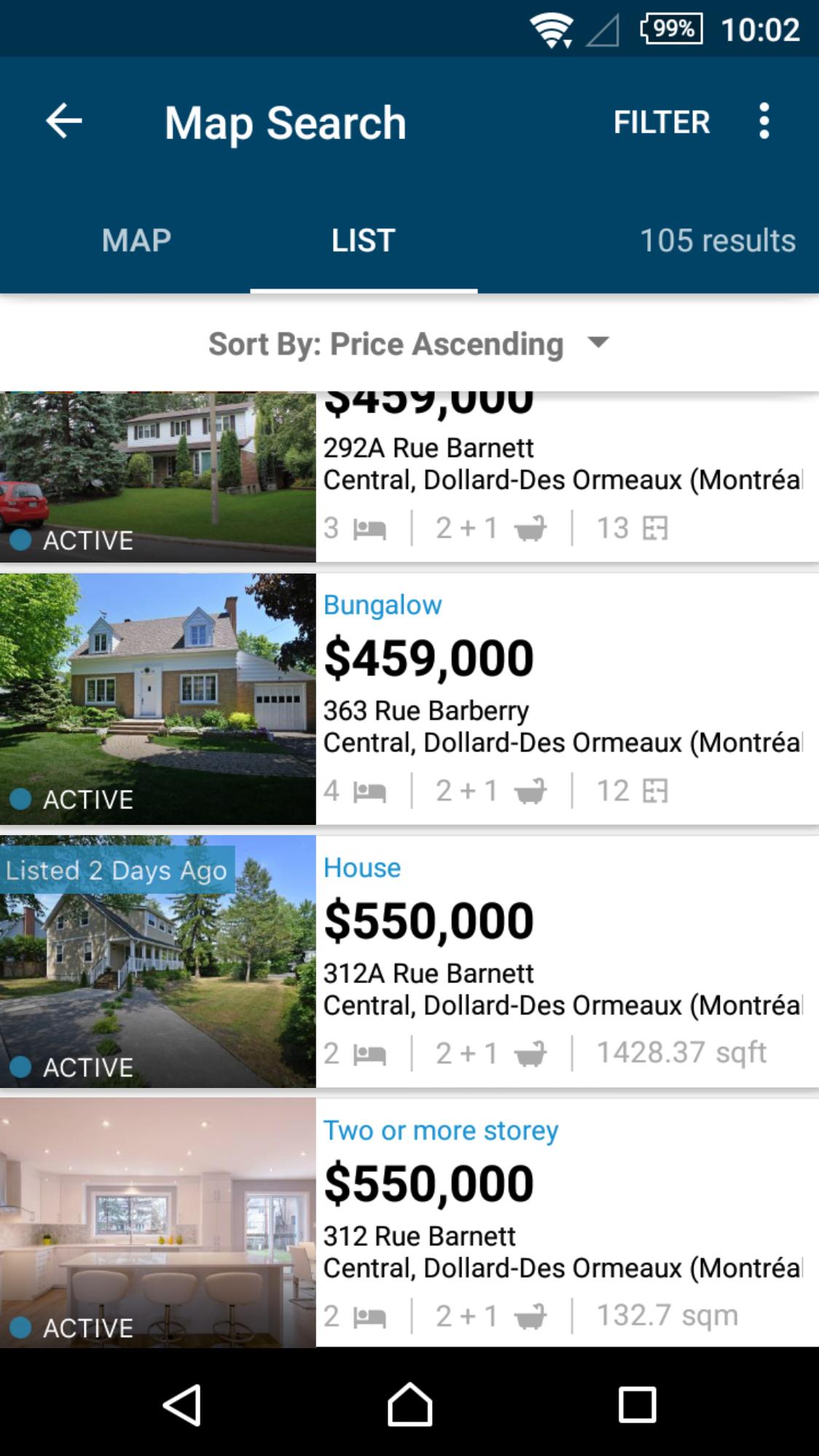This image displays several MLS listings for homes in Montreal, potentially aimed at buyers rather than renters given the high prices. At the top of the screen, there is a navigational bar with options such as 'Map Search', 'Map', and 'List', highlighted with a blue area and an arrow pointing left. The listings are sorted by ascending price.

The first home, listed at $459,000, is marked as active and has just been added to the market. It is located on RUE BARNATT street, which seems to be the common location for all the homes shown. The second property is also listed at $459,000. The third and fourth homes are slightly more expensive, each priced at $550,000 and situated on the same street. The image implies that these homes are newly listed and they all appear to be attractive options for potential homebuyers in Montreal.